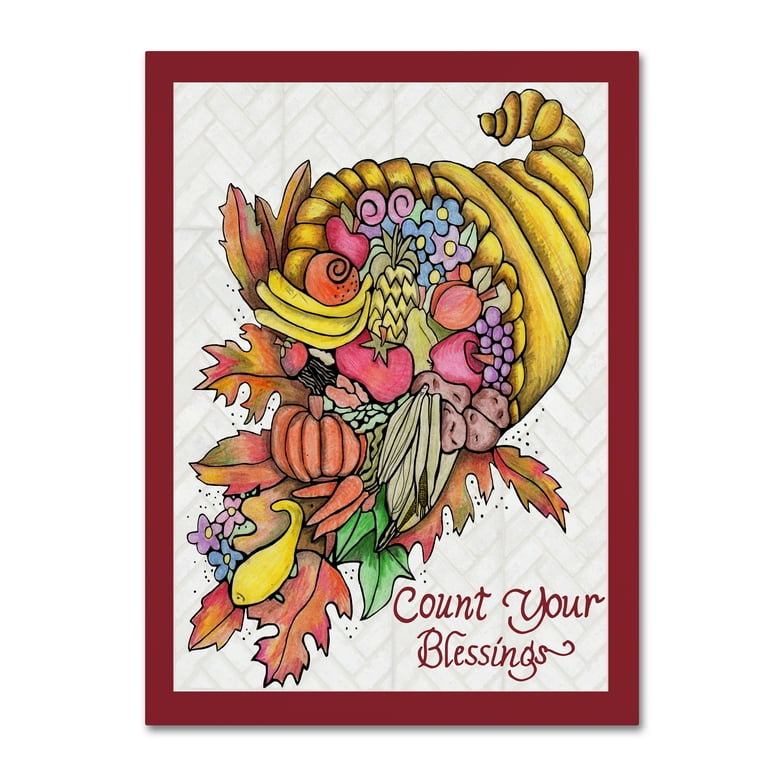The artwork depicts a festive fall or Thanksgiving-themed design, most likely intended for a garden flag or greeting card. It features a maroon border framing a white background with a subtle brick-like diagonal pattern. The focal point is a golden-yellow cornucopia spilling an abundance of autumnal harvest: vibrant fruits, vegetables, and foliage. Among the assortment, there are pumpkins, apples, bananas, purple grapes, yellow squash, ears of corn, a pineapple, and a variety of green and orange leaves. Complementing the rich cornucopia is a scattering of flowers. In the bottom right corner, in elegant red cursive, the phrase "Count Your Blessings" serves as a heartfelt reminder. The detailed and colorful composition encapsulates the essence of gratitude and abundance.